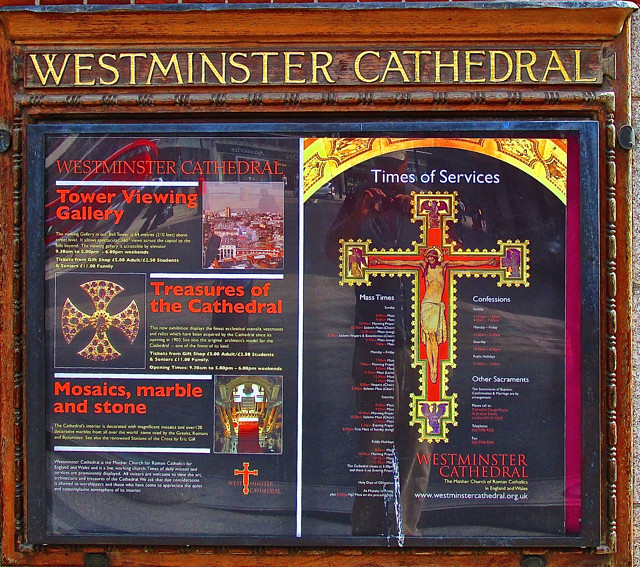The image depicts a wooden plaque encased in glass with the title "Westminster Cathedral" inscribed in gold at the top. Beneath the title, the glass cover houses an informational leaflet divided into two sections.

On the left side, the leaflet features:

- "Westminster Cathedral" at the top, followed by "Tower Viewing Gallery" in red text, and a photograph showcasing the view from the tower. Below this is some gold text providing additional information.
- The section titled "Treasures of the Cathedral" with a picture of a gold brooch next to it and further descriptive text in gold.
- The section titled "Mosaics, Marble, and Stone" in red text, accompanied by a relevant image and explanatory text underneath.

On the right side, the leaflet displays:

- An image of Jesus on the cross with the heading "Times of Services" in white.
- Detailed information about mass times, confessions, and other sacraments.
- The URL "www.westminstercathedral.org.uk" at the bottom for more information.

In the reflection of the glass cover, the photographer—a white male dressed in a blue top, khaki trousers, and a baseball cap—can be seen.